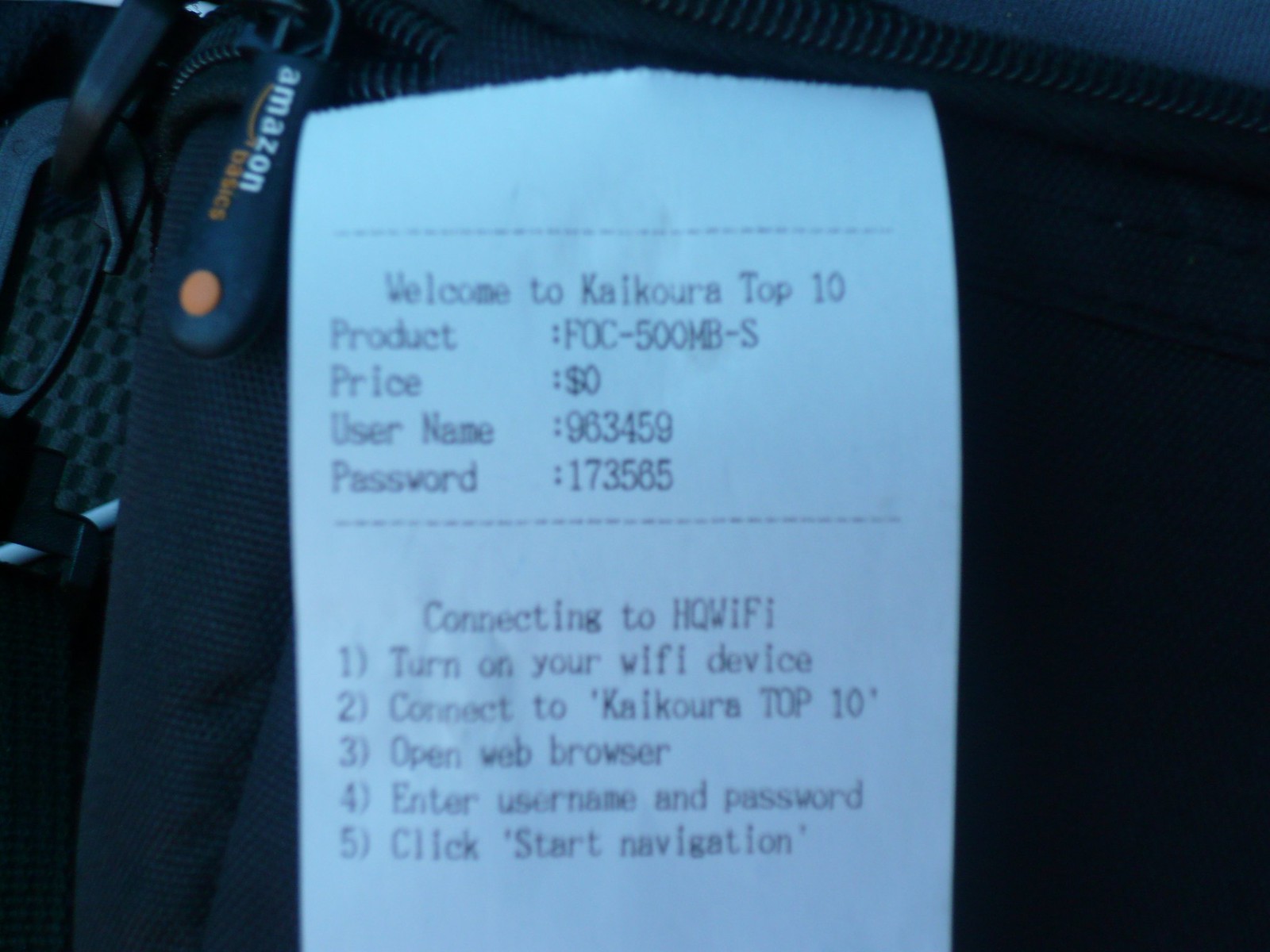The image features a receipt-like slip of paper against a very dark, nearly black background. The receipt has a white background with bluish-gray writing and highlighted details outlined by dotted lines. At the top left corner of the image, the word 'Amazon' appears in white font, accompanied by an orange button below it, all of which seem to be part of a bag, possibly suggested by visible straps or pedals on the floor. 

The text on the receipt reads: "Welcome to Calcora Top 10 Product FOC 500MB-S, Price $0, Username 963459, Password 173585," followed by instructions, "Connecting to HQ Wi-Fi: 1. Turn on Wi-Fi device, 2. Connect to Calcora Top 10, 3. Open web browser, 4. Enter username and password, 5. Click Start, Navigate."

The receipt is clearly the focal point of the image, with the rest of the background being indistinct and black.